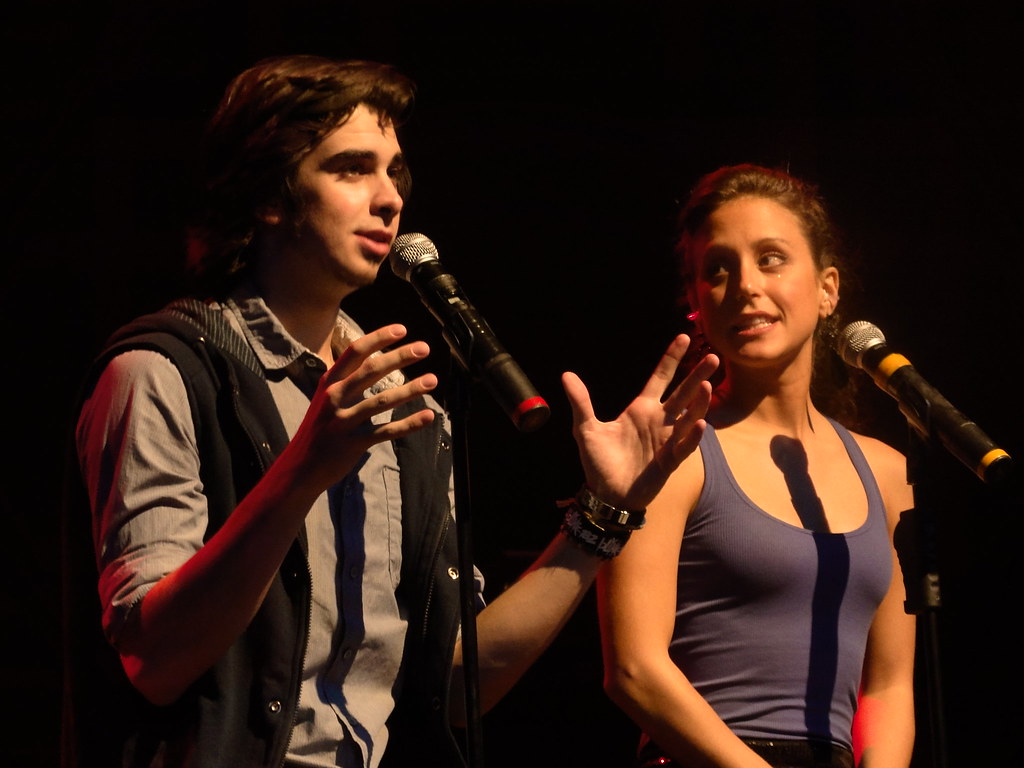In the spotlight against a completely black background, two young performers are captured from the waist up, standing side by side on stage. The young man on the viewer’s left is speaking into a large black microphone with a silver tip, mounted on a stand. He is dressed in a gray button-up shirt with the sleeves rolled up, layered under a black vest. His shoulder-length brown hair frames his olive-toned face. His deep-set eyes and thin lips are focused intently forward as his hands hover animatedly beside the microphone stand, emphasizing his speech. 

To the viewer’s right, the young woman, with whiter skin and brown hair pulled back, stands silent, her gaze fixed on the young man. She has a similar microphone placed in front of her, also black with a silver tip, but she does not appear to be speaking. She wears a blue-purple tank top and her expression is tense, revealing her teeth as if caught in a moment of grimace or contemplation. The deep blackness of the background intensifies the spotlight on the performers, highlighting the intensity of their interaction.